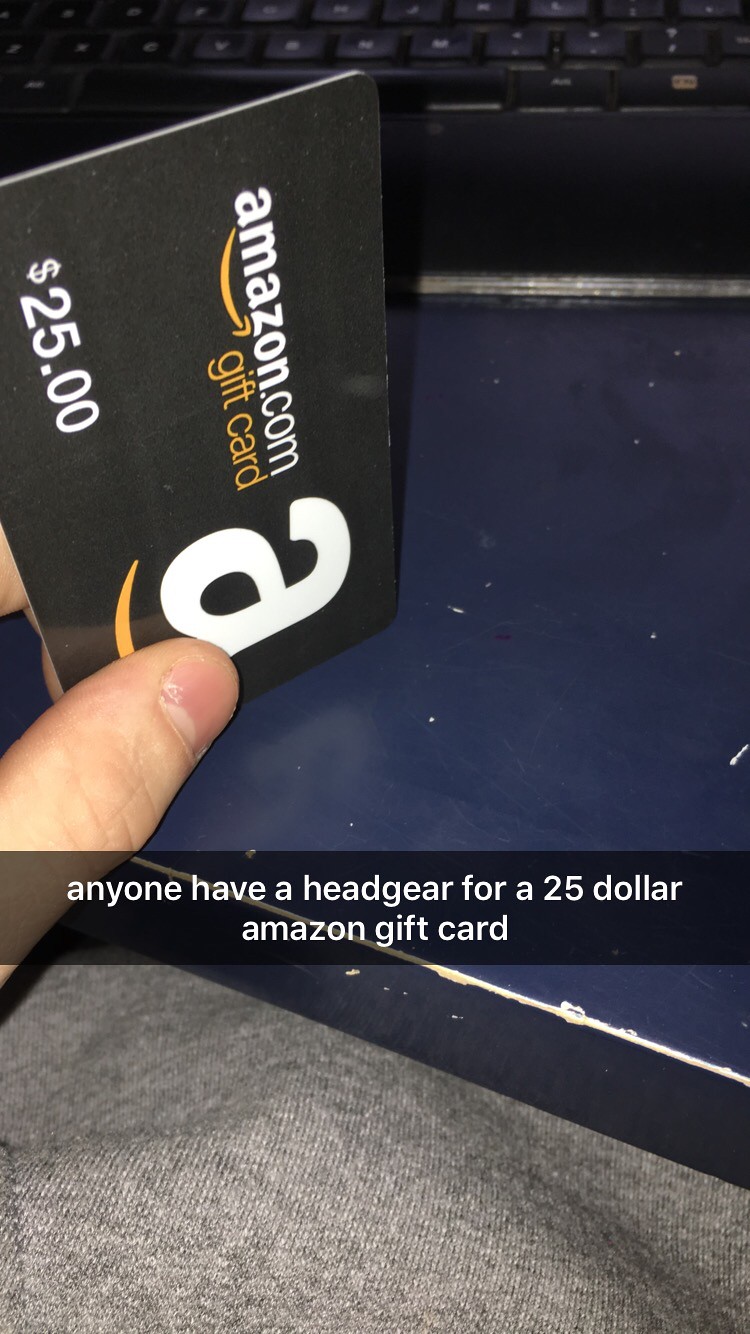In this zoomed-in image, a person is holding a black Amazon gift card worth $25 vertically between their thumb and index finger from the left side. The gift card features the text "Amazon.com" in white, a yellow arrow, the words "gift card" in yellow, and "$25" in white at the bottom, along with a large white "A" logo with a yellow stripe beneath it. Positioned below the gift card, there is a blue surface, which appears to be the top of a desk with some scuffed paint. At the very bottom of the image, a gray woven fabric is visible. In white text across the image, it reads, "Anyone have a headgear for a $25 Amazon gift card?" At the top of the photo, part of a black keyboard, including the hand rest and the first row and a half of keys, is also visible.